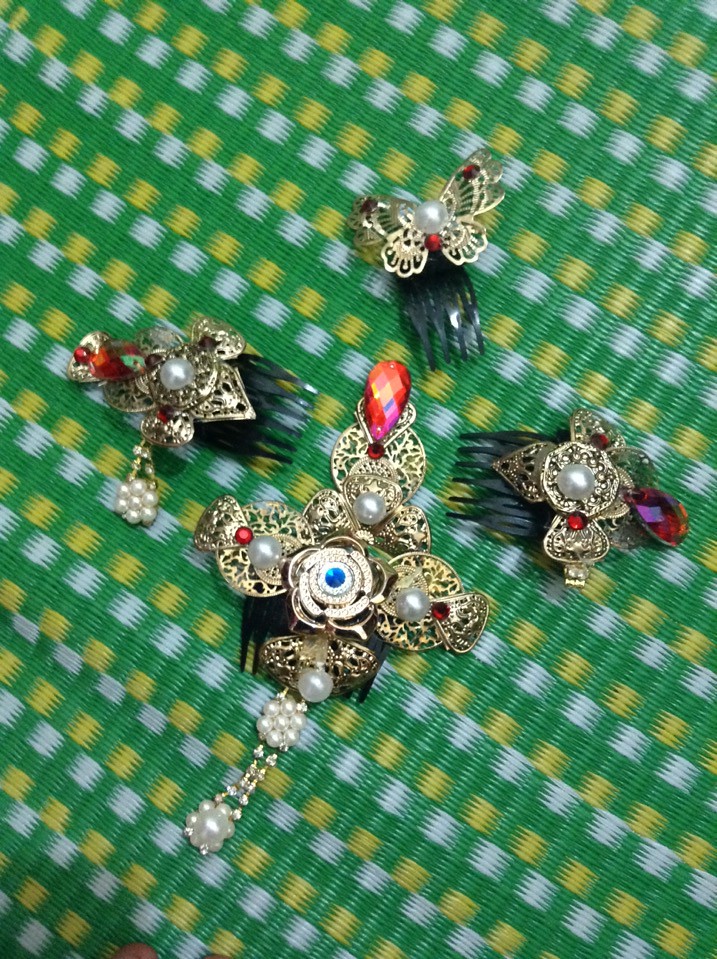This photograph showcases four ornate hair combs set against a green, white, and yellow checked tablecloth, which has a plastic, woven appearance. Each comb features intricate gold filigree designs embellished with pearls and jewels. The top comb resembles a butterfly with a pearl centerpiece and red gemstone accents. The centrally placed, largest comb has a cross-like shape, adorned with a red jewel and pearls, including dangling pearl accents, and a noticeable black comb part. The two smaller combs flanking it also display gold filigree with pearls and red gemstones. The arrangement of the combs and the detailed craftsmanship create a visually appealing composition.